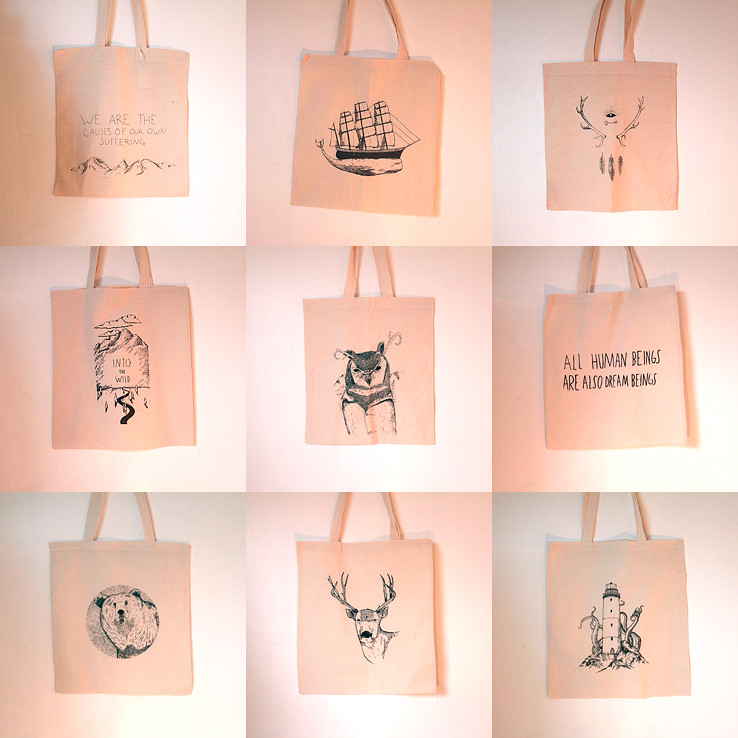The image is a 3x3 grid, displaying nine light brown tote bags set against a pink and purple background. Each tote bag features a unique design:

1. The top left tote bag displays the message, "We are the causes of our own suffering," above an illustration of mountains.
2. The next tote bag features an old ship with masts, carried by a whale.
3. The tote bag to the right shows deer antlers with feathers hanging below them.
4. The first tote bag in the second row bears the message, "Into the wild," with a pathway leading to mountains.
5. The center tote bag in the second row depicts an owl wearing a jacket.
6. The next tote bag in the second row has the message, "All human beings are also dream beings."
7. The first tote bag on the bottom row features a bear inside a circle.
8. The next tote bag in the bottom row shows an illustration of a deer with impressive antlers.
9. The final tote bag illustrates a lighthouse with a sea serpent tangled behind it, rising above it.

Each tote bag is meticulously designed to convey a unique artistic expression.